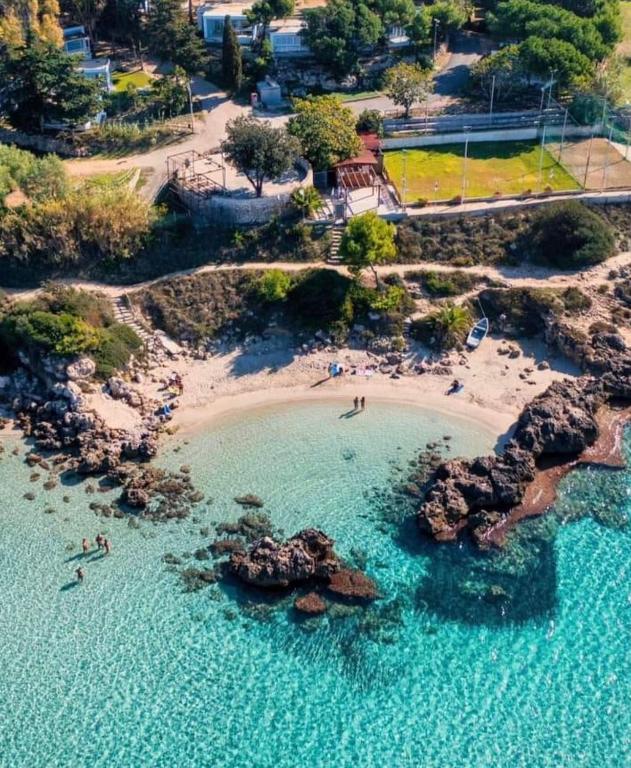This vivid aerial view captures a stunning landscape featuring a clear, soft turquoise body of water, edged by a sandy beach and surrounded by an array of rocks and small shrubs. The image showcases a serene daytime scene where a couple of people are seen standing at the water's edge, while others are lounging on towels on the sand. To the left, steps lead down to a distinct pool of water, which is encircled by jetties forming a unique geometric shape. A walking path and a grassy ledge provide additional access to the beach, with further pathways and a quaint bridge visible in the upper section. The background reveals a park-like area with a small green grass field, scattered with trees and bushes, and dotted with a few houses and buildings in the distance. The clarity of the water and the harmonious blend of natural and man-made elements suggest this could be a picturesque tourist destination or a resort, offering a beautiful and inviting escape.